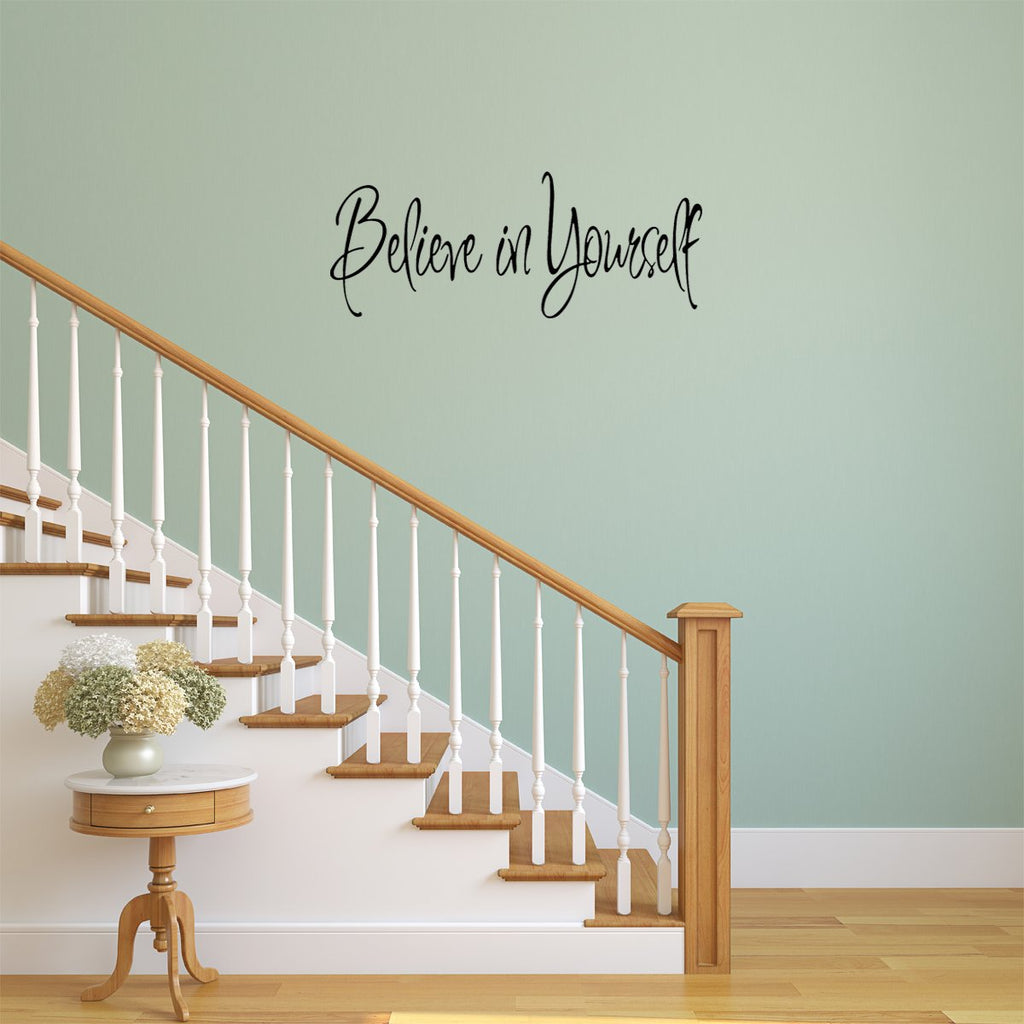The image depicts a modern two-story home interior, focusing on a staircase that ascends from the center of the frame to the upper left. The staircase features light-colored wooden steps, accented by a white banister. Across from the staircase, a prominent light green wall is adorned with the inspiring phrase "Believe in Yourself," painted in large, clear letters. At the base of the stairs, there's a small, round, light wood table with a white marble top. On this table sits a white vase holding big, rounded, green and white flowers. The overall aesthetic is clean, modern, and minimalistic, with a hint of computer-generated perfection in the portrayal of the home's new appearance. The light wood flooring complements the staircase and table, enhancing the serene and inviting ambiance of the interior.